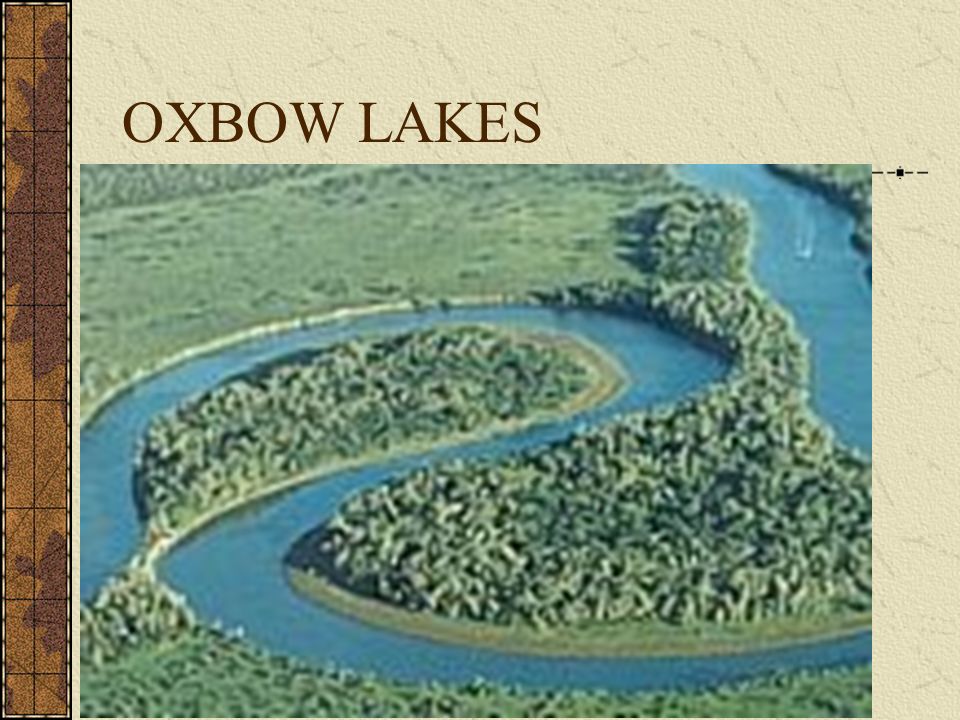The image features a vibrant aerial photograph of Oxbow Lakes, clearly labeled in bold brown text at the top of the image. The photograph depicts a lush, green area intersected by a meandering river, which starts from the left-hand side, loops around curving like the letter 'E' and moves off to the right-hand side. The waterway forms natural semicircles and a full circle around green islands covered in grass, bushes, and small trees.

Surrounding the image is a light tan or parchment-like border, reminiscent of a scrapbook or old map. This adds a vintage feel and provides a contrast to the lush greens and blues of the photograph itself. On the left side of the image, there's a distinctive vertical brown strip, detailed with leaf patterns and thin black boxes, enhancing the visual frame. This strip appears to be part of the graphical design, giving the impression of a formal presentation slide. The overall composition, including the marbled off-white background, accentuates the serene beauty of the Oxbow Lakes, making it a visually captivating snapshot of this natural phenomenon.